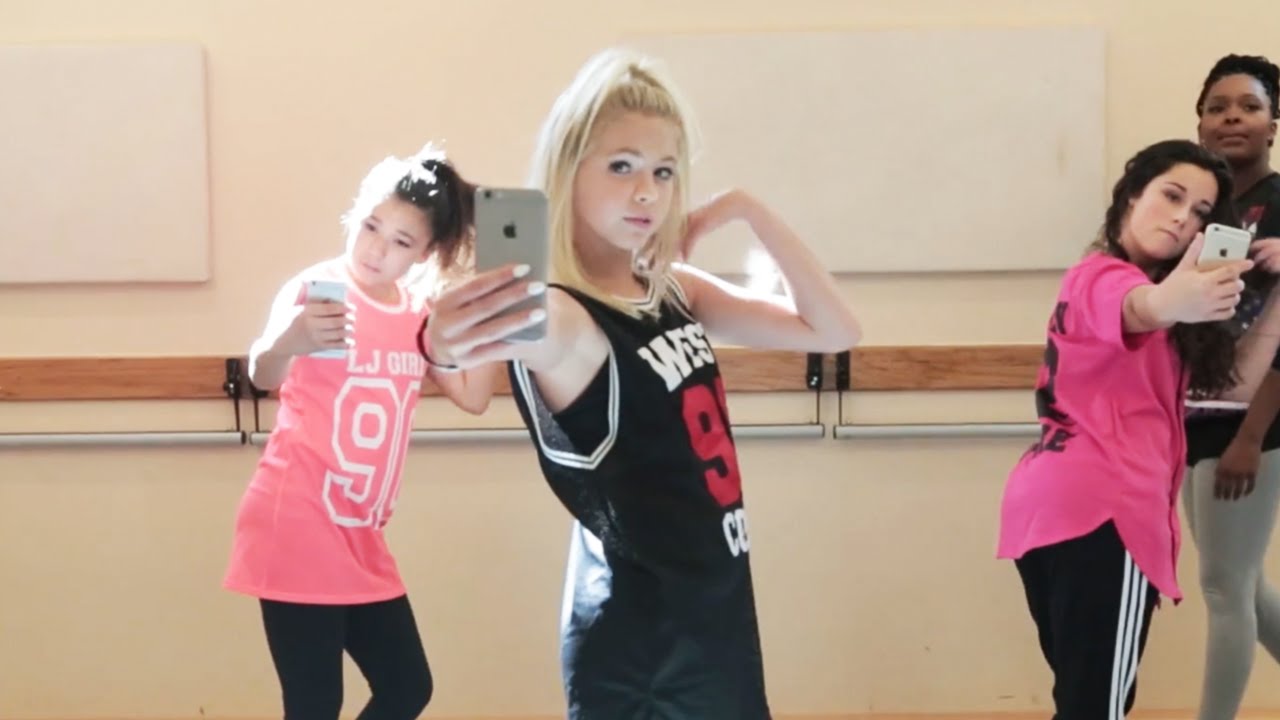The photograph depicts a dance class scene featuring three preteen girls and an adolescent boy, all in a dance studio. The girls are dressed in athletic attire: the central girl, who is blonde with a high ponytail and white nail polish, wears a black tank top with "West 9" emblazoned on it and black leggings. Her tank top has white trim on the armholes and neck. To her left, a brunette with her hair in a brown ponytail, is outfitted in a pink tank top with large white "90" graphics, paired with black leggings. She takes a selfie, holding a silver iPhone in her right hand. To the right of the blonde girl is another brunette, her hair braided back, dressed in a dark pink tank top with black lettering and black leggings. She leans her head on the chest of the boy next to her, capturing a selfie with her iPhone. The boy standing beside her wears gray track pants and a black t-shirt. Behind this group, a Black woman in gray leotards and a black shirt walks through, observing the scene, possibly the dance instructor. The dance studio features a beige wall, a ballet barre, and two white wooden blocks resembling canvas frames. The scene captures a moment of focused self-expression as they take selfies, seemingly bonding through the shared activity.